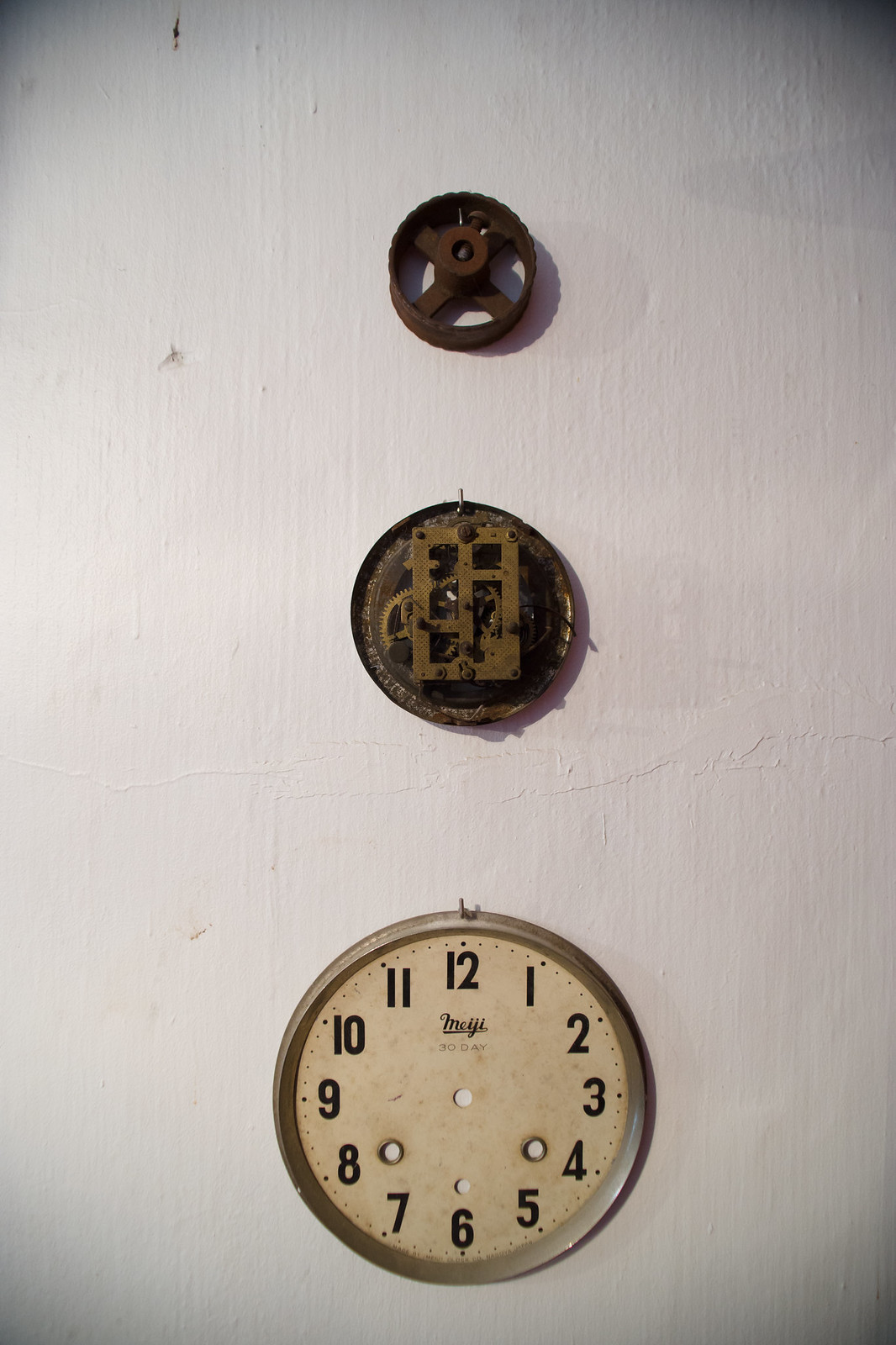This detailed photograph showcases an old vintage clock that has been meticulously taken apart and displayed across a white, textured surface. The image is rendered with a vignette effect, darkening the corners and illuminating the center. 

At the bottom, we have the face of the clock, which features bold black numbers ranging from 1 to 12. The clock face is noticeably weathered, exhibiting yellowing and browning against its light off-white background. Prominent in the center of this clock face is the brand logo, labeled as "M.I.J.I," along with four holes intended for rivets to secure it to the clock's internal structure. A silver rim encircles this component, adding to its vintage charm.

Positioned in the middle is the clock's mechanical core, a somewhat larger circular piece containing intricate gears and other machinery. This component is crucial to the clock's function and exhibits a lighter brown hue with visible signs of aging.

At the top, we find a smaller metal gear wheel that also has a circle-on-X design, browned and rusty from age, vividly capturing its historical essence.

The entire setup is placed on a white-painted surface with visible lines and textures, providing a rough but suitable backdrop that further enhances the image's nostalgic tone. A bright white light shines from the left, accentuating the details of these meticulously arranged clock pieces.